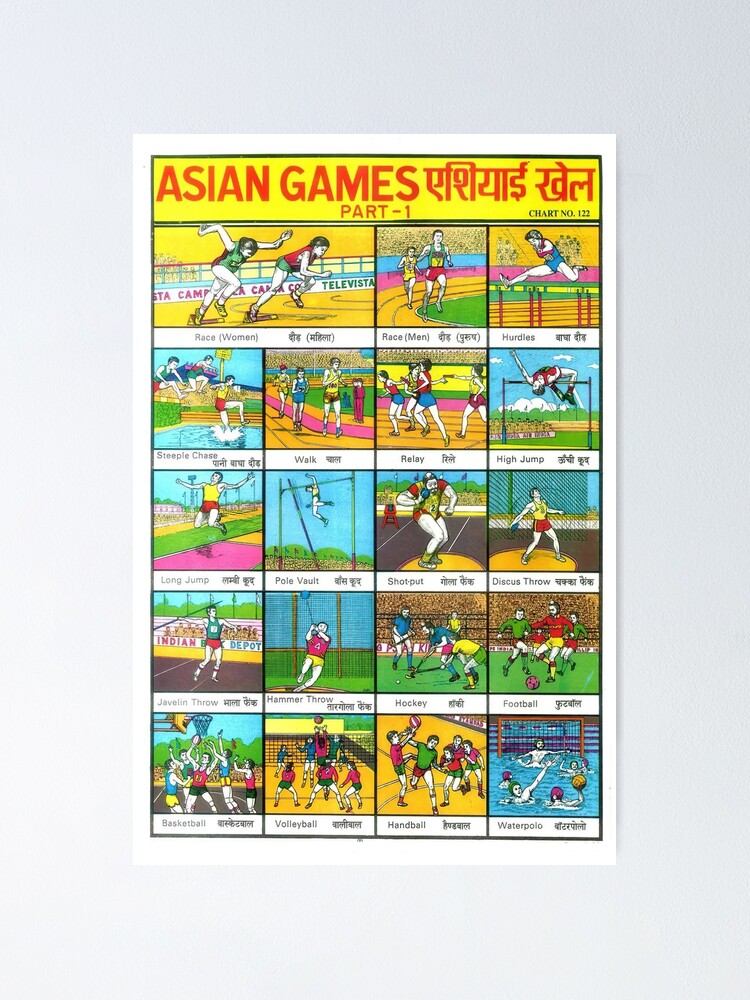The image appears to be a poster-like chart with a light blue, textured background resembling a wall. It is laid out in a grid format with illustrations, similar to a comic strip spanning three to four squares across five rows, resembling the size and orientation of an A4 page. At the top, bold red text reads "Asian Games Part One" with "Chart Number 123" in black text to its right. Above this, there is text written in an unrecognized foreign script. The chart consists of various animated illustrations, each representing different sports, including volleyball, soccer, high jump, basketball, swimming, women's race (twice as long as the others), hurdles, relay, walking, steeplechase, pole vaulting, long jump, javelin throw, hammer throw, football, hockey, and water polo. The consistent, detailed graphics suggest these illustrations might have been computer-generated, portraying people actively engaged in these sports.